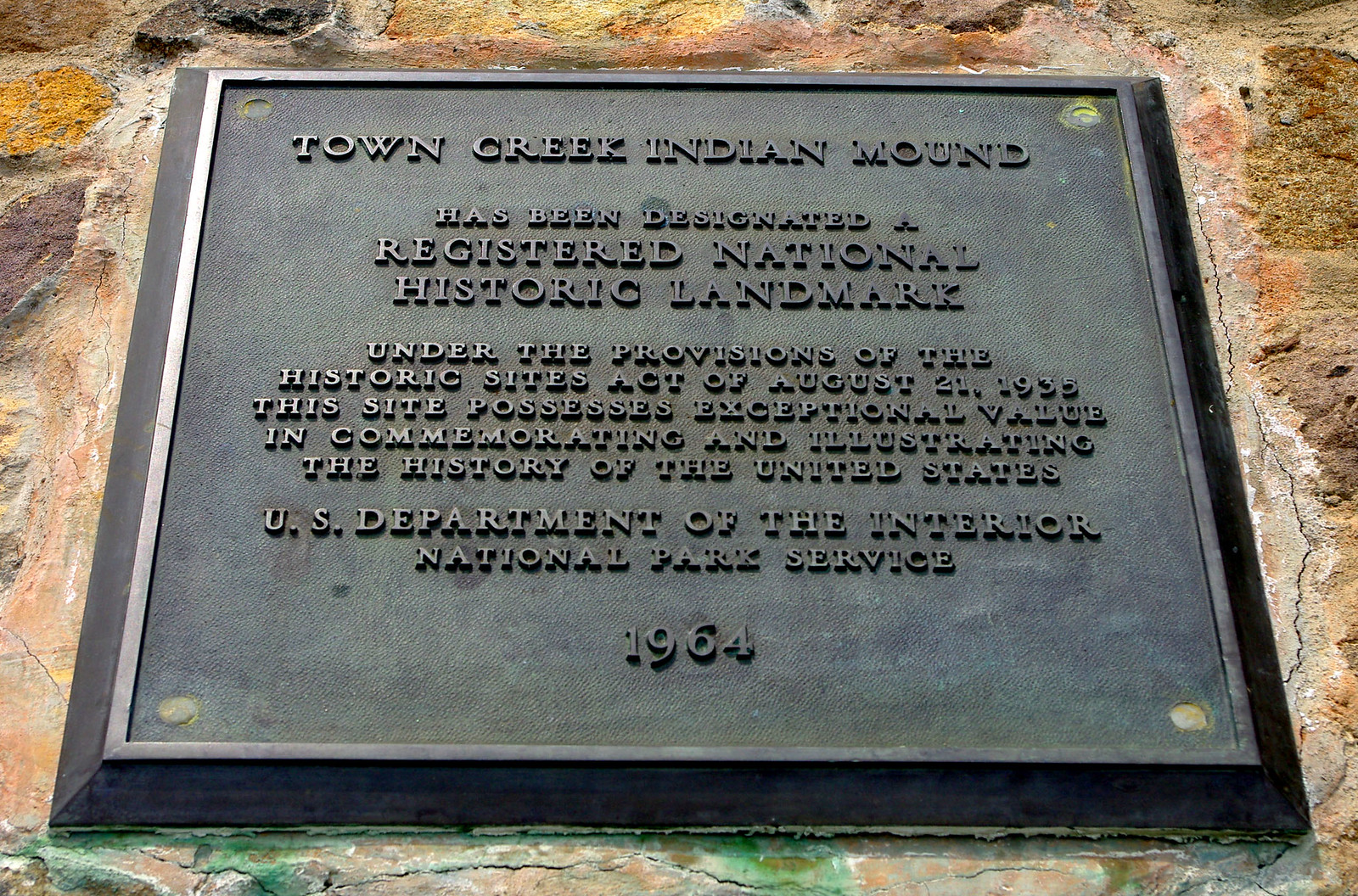The image features a detailed black plaque with embossed golden text, mounted on a weathered stone wall comprised of orangey-yellow-beige and greenish moss-covered stones. The plaque has a silver border and is secured to the wall with four screws, one in each corner. The plaque reads "Town Creek Indian Mound" and declares the site as a registered National Historic Landmark under the provisions of the Historic Sites Act of August 21, 1935. It states that the site possesses exceptional value in commemorating and illustrating the history of the United States. The plaque is designated by the U.S. Department of the Interior National Park Service in 1964. The stones surrounding the plaque are of varying colors and appear cracked and aged, reinforcing the historic and venerable nature of the site.